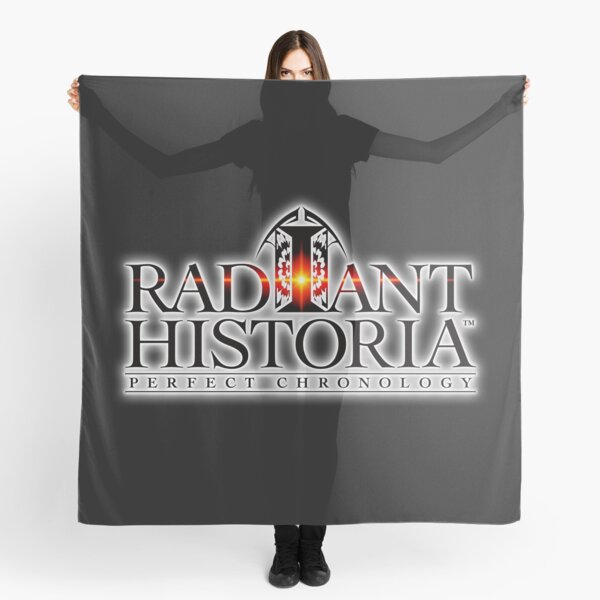In this photorealistic image set against a white background, a slim young woman with long, straight brown hair extends her arms to hold up a sheer, semi-transparent gray fabric in front of her face and body. Only her expressive eyes and forehead are visible above the fabric. She is dressed in a black t-shirt, tight black pants, and black boots. The fabric, which resembles a flag or cape, prominently displays the logo "Radiant Historia Perfect Chronology." The letter 'I' in "Radiant" is uniquely styled to resemble a stained glass window featuring a sunbeam effect through the word, giving it a bright, radiant appearance. Her fingertips can be seen gripping the upper corners of the fabric, adding a touch of human detail to the overall composition.